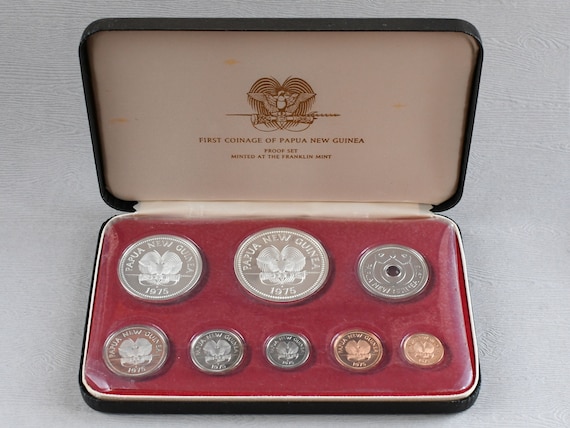This photograph features a collector's set of eight coins from Papua New Guinea, minted in 1975, housed in an open black case with a red felt interior. The inside cover of the case displays the text "First Coinage of Papua New Guinea Proof Set, Minted at the Franklin Mint." The coins vary in size and color, predominantly silver and a few with a copper-like appearance. One of the coins has a hole in the middle. The coins are arranged neatly with inscriptions visible on some, denoting "Papua New Guinea 1975." The top of the case, which is black on the outside, features a small image and additional unreadable text beneath the main inscription.